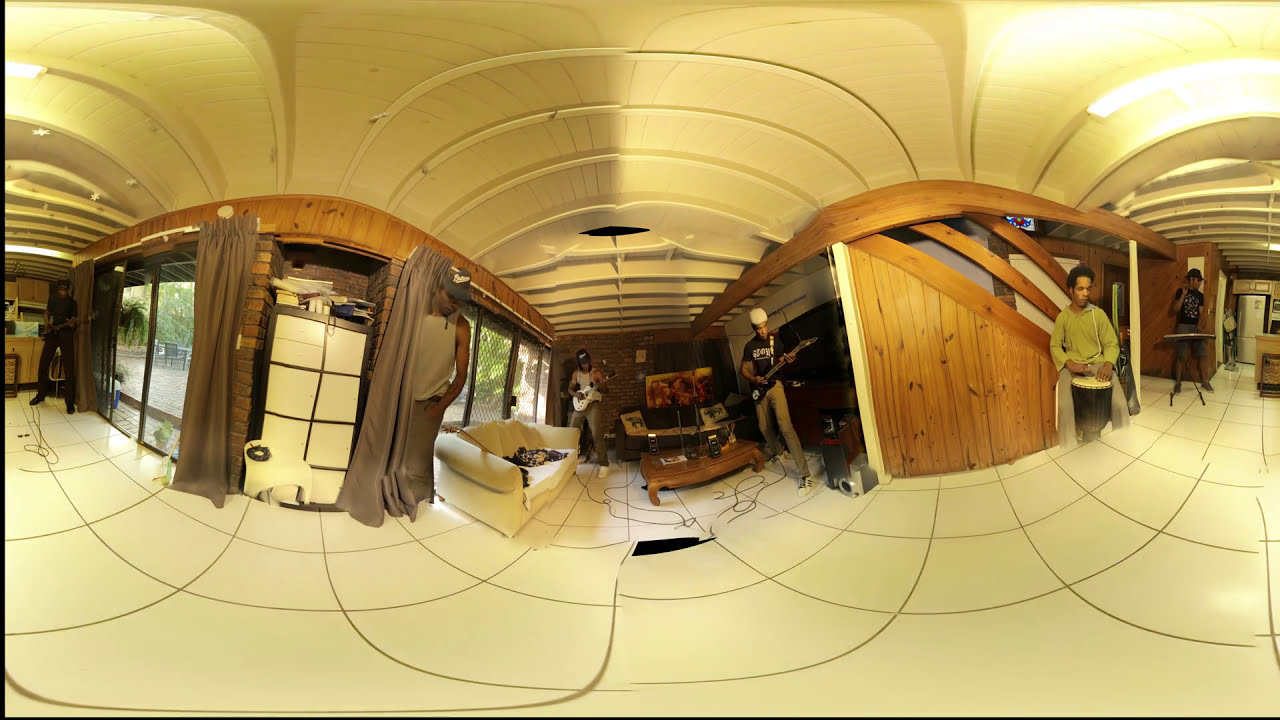The image depicts the interior of a building featuring multiple musicians seemingly in practice, and it's stylized with a wavy, distorted perspective that makes it appear as though the floor and walls are moving. The scene is divided into three parts, with distinctive elements in each section. The top and bottom margins are adorned in gold, with gold archways connecting different parts of the room. 

In the left section, a guitarist dressed in black is positioned in the back corner near a sliding glass door, flanked by open dark brown curtains. The middle section features two guitarists standing at opposite ends of the room: one in a white tank top with a white guitar and black hat, and another in a black shirt and khaki pants with a black guitar and white hat. Between them is a brown coffee table, and against the left-side window stands a white couch. Nearby, a idle person stands next to the sliding glass door.

In the right section, a person in a long-sleeved green shirt and gray bottoms is seen playing a hand drum, with the lower part of their legs cut off in the frame. Another musician, wearing a black T-shirt and gray shorts, is playing a keyboard against a brown wall. The room itself has a white floor and ceiling, both featuring black curved lines that add to the distorted visual effect. The walls are trimmed with wood, enhancing the warm ambiance of the space.